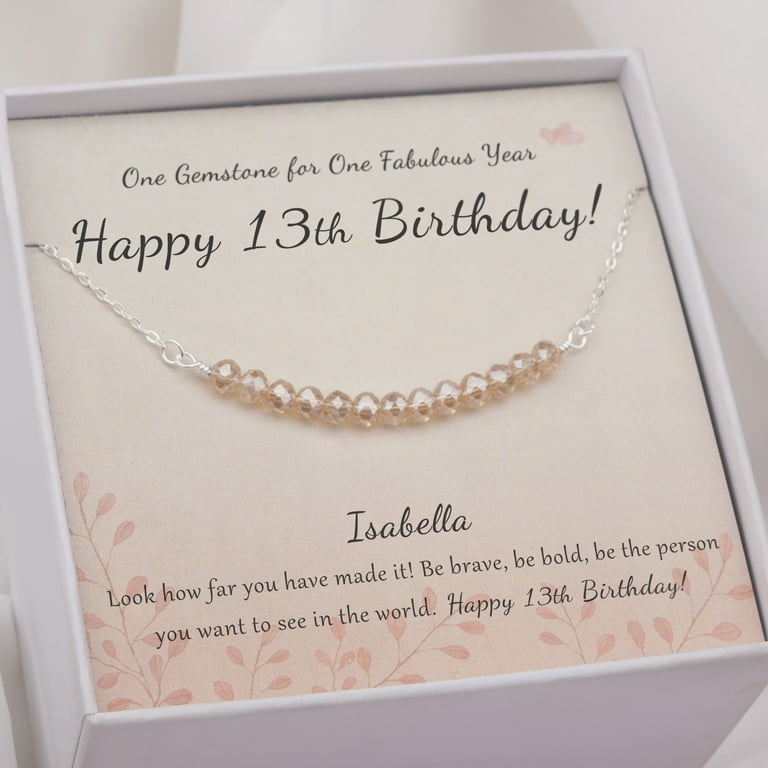This detailed photograph captures a heartfelt gift for a child's 13th birthday, set against a pristine white background. The centerpiece of the image is an open white jewelry box, prominently displaying a thoughtful message on a peach-colored piece of stationery adorned with delicate, watercolor-style leaf stamps in shades of red and light pink. The card reads, "One gemstone for one fabulous year. Happy 13th birthday!" in elegant black cursive, with an exclamation mark emphasizing the celebratory note. Draped beneath the text is a sophisticated pearl bracelet, each of its 13 pearls symbolizing a year, and the bracelet is suspended by a silver chain adding a touch of grace to the presentation. Further down the card, also in black cursive, is the name "Isabella," accompanied by an inspiring message: "Look how far you have made it. Be brave, be bold, be the person you want to be in the world. Happy 13th birthday." To the right of the text, there is a small, charming butterfly, enhancing the whimsical nature of the gift. The entire display exudes a sense of love and encouragement, perfect for marking such a significant milestone in a young person's life.